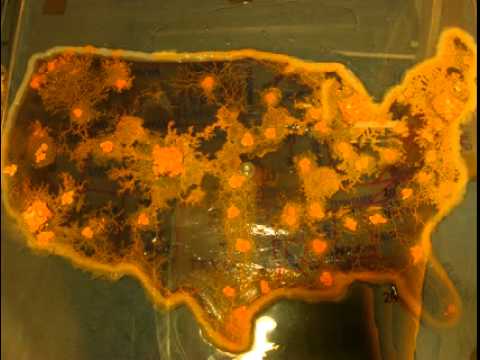The image depicts a small, low-quality photograph of an art piece showcasing the outline of the United States. The central shape of the U.S. is prominently featured with a distinctive orange hue interspersed with deeper shades of brown and gray. The outline is framed by a yellowish-orange border, and the backdrop is a greenish color, giving the impression of a painted or hand-crafted artwork. The United States map is perfectly positioned in the center of the composition, possibly displayed on a table, as suggested by the visible light reflection beneath the Texas area. The piece is lit from below, highlighting its intricate details, yet there is no time, date stamp, text, or labeling to offer additional context. The setting remains ambiguous, leaving it open to interpretation as either a museum exhibit or a personal art project.